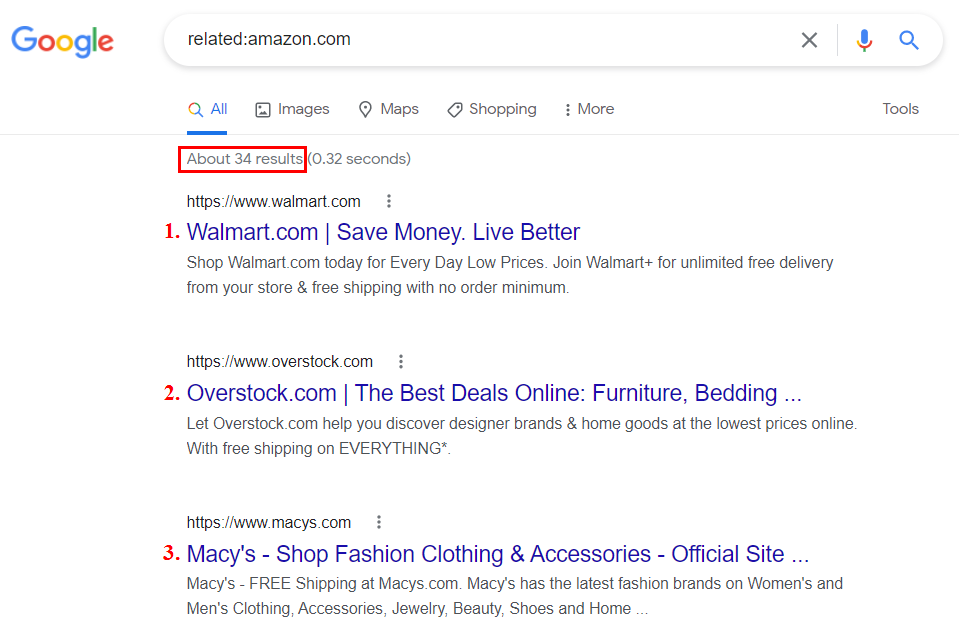A detailed caption for the image based on the provided description could be:

---

The image shows a Google search results page with the query "related:amazon.com" displayed. This specific search yields 34 results, prominently highlighting major online retailers similar to Amazon. Featured among the results are Walmart, Overstock, and Macy's, each with their respective slogans: "Save Money. Live Better." for Walmart, "The Best Deals Online" for Overstock, and "Shop Fashion, Clothing, and Accessories" for Macy's. The page maintains the traditional Google layout, with a white background and black and blue text. There is an editorial box around the text "about 34 results," emphasizing the total count of search outcomes. This highlighted box indicates careful editing, possibly to draw attention to the search effectiveness. The purpose of this search is to illustrate how Google interprets queries to find websites comparable to Amazon, showcasing other major e-commerce platforms as a result.

---